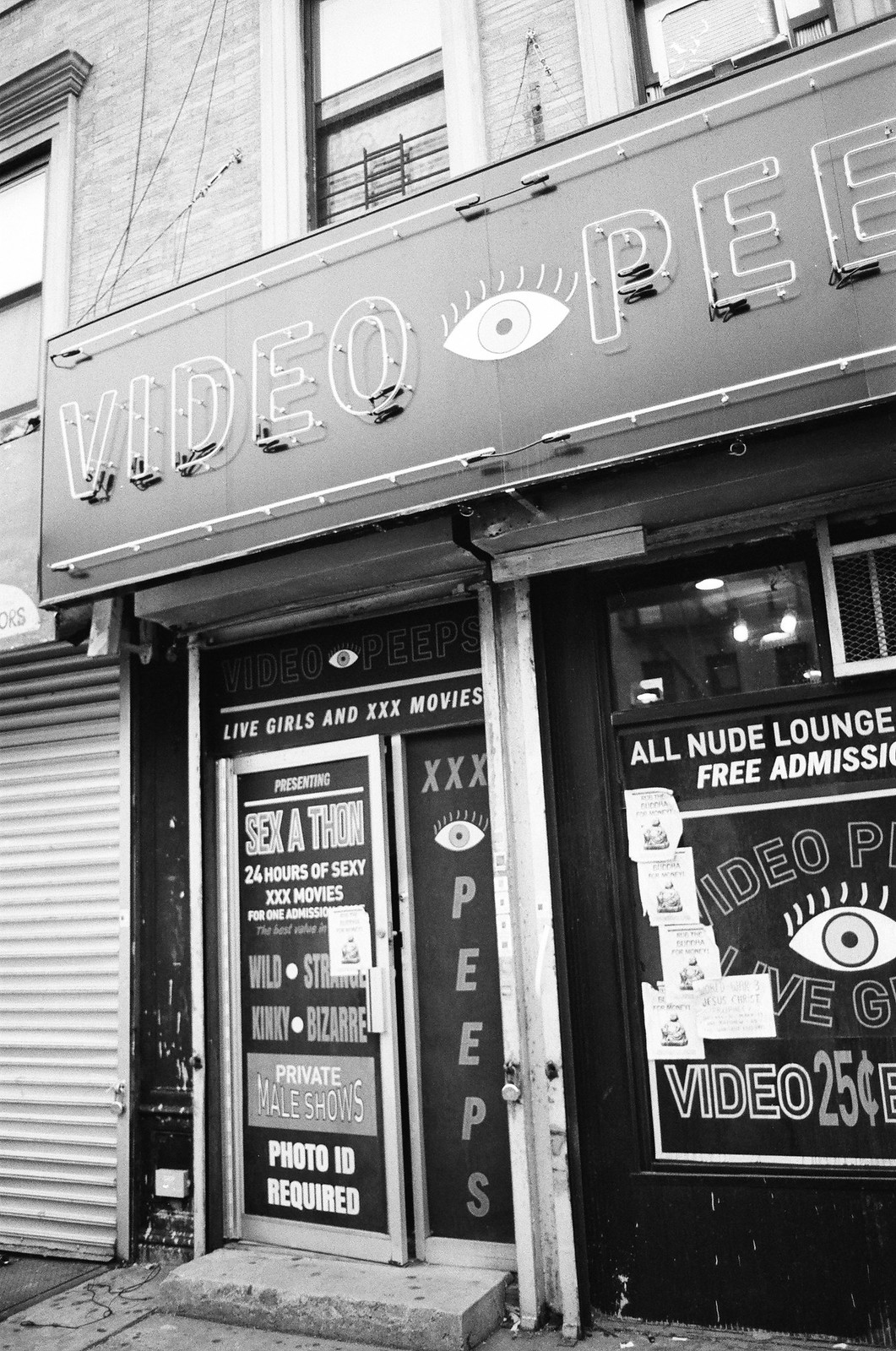This detailed black-and-white photograph captures the front of a seedy adult entertainment store. At the top of the doorway, there's a banner reading "VIDEO PEE" with an eyeball logo, suggesting "video peep show." The silver-framed door below the sign features numerous provocative advertisements, including "Live Girls" and "XXX Movies." A bold statement announces "Presenting Sex-a-thon: 24 Hours of Sexy XXX Movies," followed by "Wild, Kinky, Bizarre" and "Private Male Shows" with "Photo ID Required" at the bottom. To the right of the door, the branding continues with "XXX" and "PEEPS" alongside the eyeball logo. The right window is conspicuously covered, bearing the notice "All Nude Lounge, Free Admission." Further down, partially visible text states "Video 25 cents," with various flyers plastered around. The image suggests a run-down establishment, accentuated by the stark, monochromatic tone and a single concrete step leading up to the entryway.